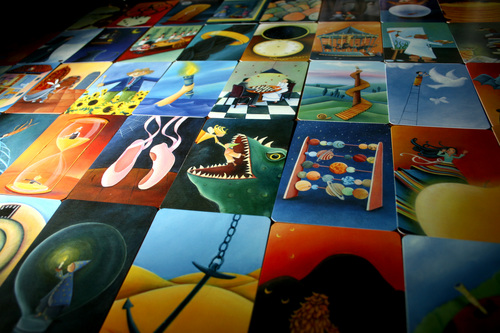This image depicts a colorful and surreal collection of Dixit game cards arranged in a grid-like formation, almost resembling a tiled wall. The cards, each in a rectangular shape similar to playing cards, are tightly packed together, creating a vivid and eclectic montage. Notable illustrations on the cards include an hourglass with an orange background, an abacus featuring planets, an anchor set in a desert landscape, and ballet shoes poised on their toes. Other remarkable images feature a green lizard with its mouth wide open, seemingly engulfing two small people, a stopwatch, and a girl's outstretched arm reaching for a dove at the top of a staircase. Also present are a wizard holding a candle, a person half-submerged in the sea clutching a torch, a dark mountain set against a red sky, a field of sunflowers with a scarecrow, and a fairy rescuing someone. The surreal and imaginative artwork of these cards aligns with the descriptive nature of the Dixit game. An angled view reveals multiple rows, while a black vignette frames the entire ensemble, enhancing the dramatic presentation of this diverse collection.